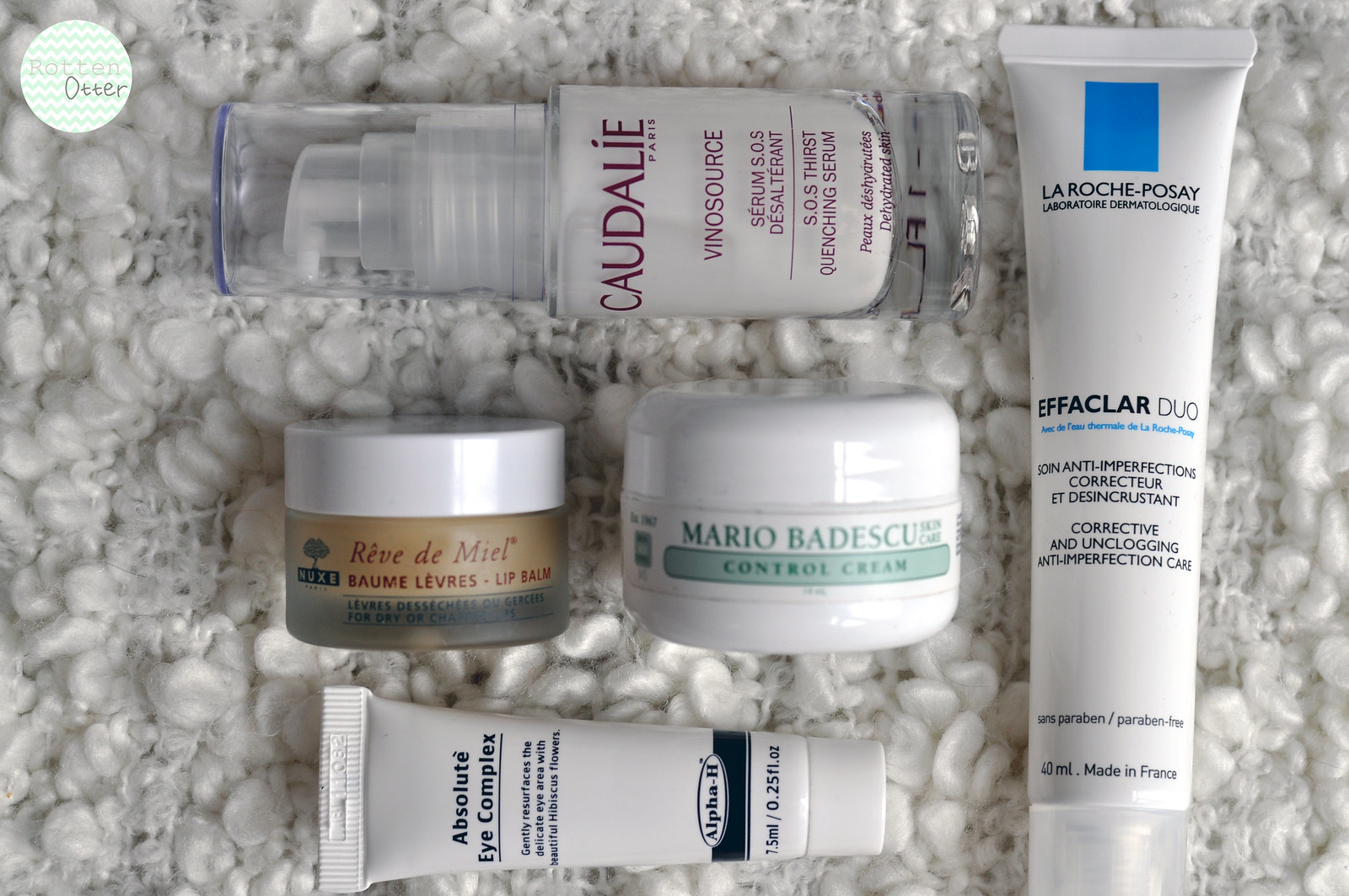The image depicts a box filled with packing peanuts at the bottom, showcasing a variety of skincare products. In the upper left-hand corner, "Rotten Otter" is labeled. 

- A jar labeled "Caudalie Vinosource SOS Thirst-Quenching Serum" is prominently situated. 
- Beneath it, there is a container of "Revlon Balm of Red Lip Balm."
- Next to that, a tube labeled "Mario Badescu Control Cream" for skincare is visible.
- Below that, the label reads "Alpha-H Absolute Eye Complex," containing 1.5 ml.
- To the right, there is a larger product with "La Roche-Posay" printed along with a blue square above its black lettering. The label details "Effaclar Duo [+] Anti-Imperfection Corrector," describing it as a "Corrective and Unclogging Care" in both English and French. It specifies a volume of 40 ml and notes that it is "Made in France."

These items are neatly displayed on top of the packing peanuts, clearly arranged for view.